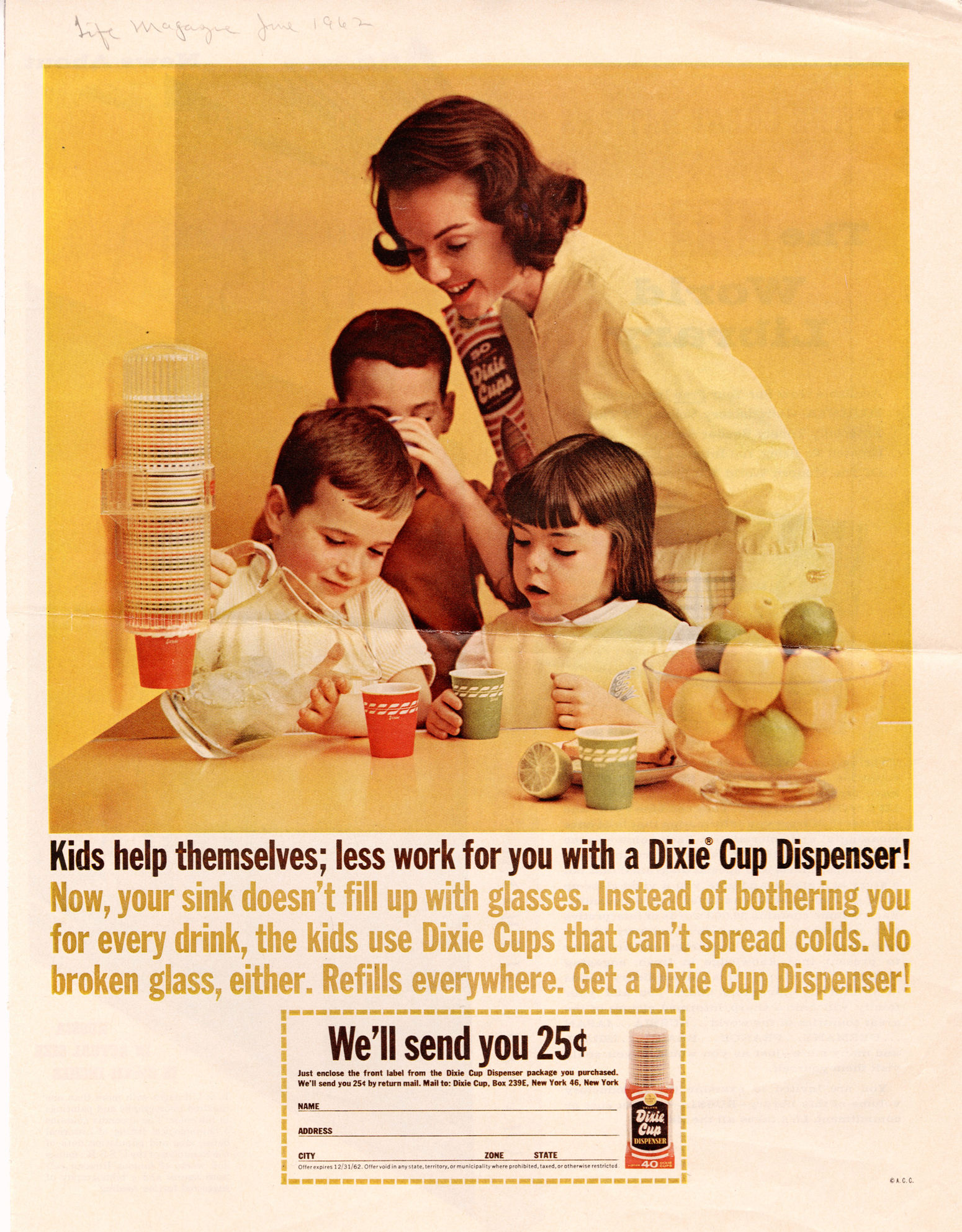The vintage magazine advertisement, from the fifties or sixties, features a vibrant indoor setting with a yellow background. At the center is a color photograph of a smiling young white woman in her thirties with short brown hair grazing her neck, and dressed in a classic white shirt. She is leaning over a counter or table, engaging with three children.

The child on her left is a small boy in a red shirt, drinking from a Dixie Cup. To his right, another young boy, around five or six years old, dressed in a white shirt, is pouring liquid from a clear pitcher into a Dixie Cup. Further right, a little girl, of similar age to the younger boy, is wearing a yellow jumper over a white shirt and holding a green Dixie Cup. She has long brown hair with bangs.

Mounted on the wall to the left of the children is a plastic Dixie Cup dispenser filled with a sleeve of numerous Dixie Cups. On the counter to the right, there is a clear glass bowl brimming with lemons and limes, one of which is cut open, and a green Dixie Cup is placed in front of it.

The background of the magazine page is beige. Below the photograph, brown lettering announces, "Kids help themselves, less work for you with a Dixie Cup dispenser." This is followed by a yellow text block reading, "Now your sink doesn’t fill up with glasses. Instead of bothering you for every drink, the kids use Dixie Cups that can’t spread colds. No broken glass either. Refills everywhere." 

At the bottom of the advertisement, a dashed-line coupon offers "We'll send you 25 cents." The coupon has spaces for a name, address, city, zone, and state, highlighting its vintage nature by omitting a zip code, and provides mailing information to Dixie Cup in New York.